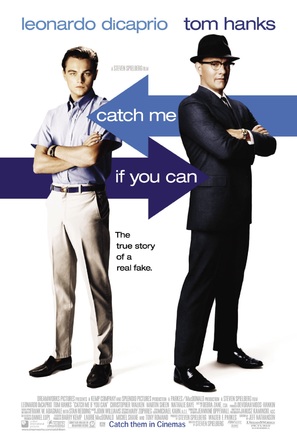This detailed movie poster features two prominent actors, Tom Hanks and Leonardo DiCaprio. Positioned centrally, the poster showcases Tom Hanks standing on the right, donning a black suit, black pants, black shoes, a black hat, and glasses. Leonardo DiCaprio is on the left, wearing a short-sleeve button-down shirt, white pants, a belt, and black shoes. Both actors are depicted with serious expressions; DiCaprio with his light brown hair and Hanks slightly turned to the side. Above DiCaprio's head, his name is boldly displayed, while Hanks' name appears above him. The poster prominently features two arrows layered behind the actors: a light-colored arrow pointing to the left with the text "Catch Me," and a darker blue arrow pointing to the right with "If You Can" written in white letters. Below these images, the tagline reads, "The True Story of a Real Fake." Near the bottom, smaller, unreadable text is present, with the larger, distinct instruction "Catch Them in Cinemas" emphasizing the movie's theatrical release.